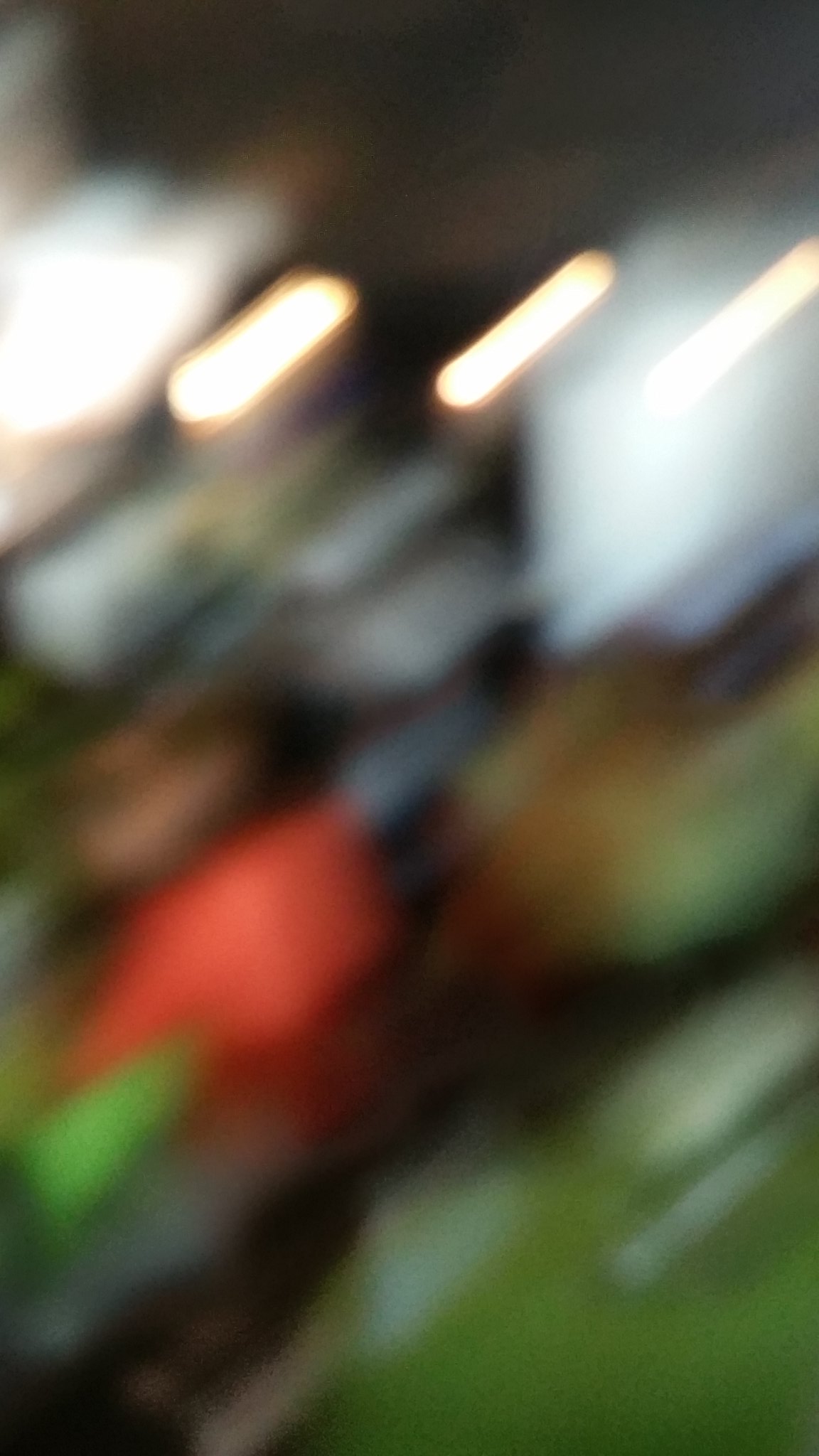This is a blurred, difficult-to-decipher vertical photo. About one-third down from the top, diagonal streaks of light, possibly from headlights or street lamps, stretch from the lower left to the upper right. Below these streaks is a splotch of red that seems to depict a person, potentially wearing a red or orange life jacket, set against a backdrop of green. The details are indistinct, making it hard to provide a definitive description. Additional large white blobs across the top serve as a background to the light streaks, adding to the photo's enigmatic quality.